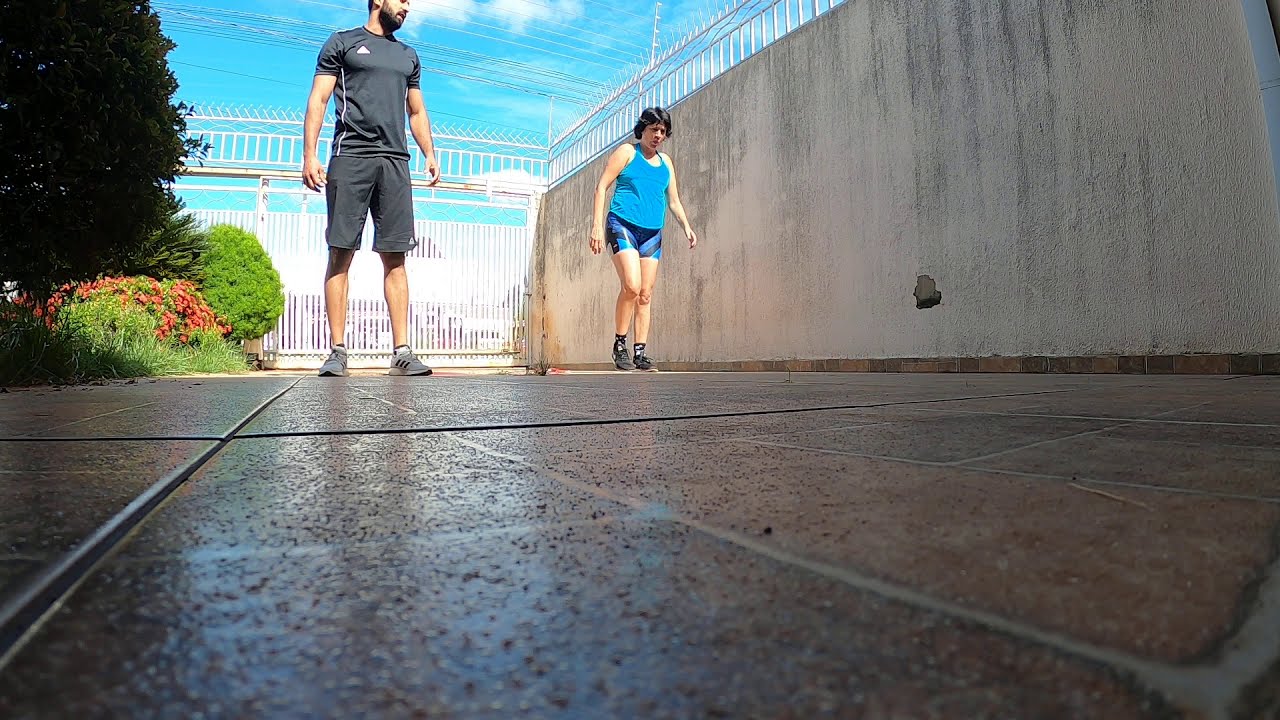In the image, there are two people standing on a ceramic-tiled walkway, with tiles held together by gray-colored grout. On the left side, a man stands facing forward, his head slightly turned to the right. He is wearing a black short-sleeved t-shirt, black shorts, gray tennis shoes, and has a full beard. Next to him, on the right, is a woman with short black hair that reaches just over her ears. She is wearing a blue tank top, blue shorts, and black shoes. Both individuals are Caucasian and appear to be either older or middle-aged.

To the far right of the scene is a gray and white concrete wall, featuring a circular hole that looks like it was punched in. Another similar hole is located near where the woman is standing. At the top of this wall is a white metal barrier. Behind the pair, there is another barrier made of white metal pipes.

On the far left side of the image, there is a dark tree with a green, globe-shaped shrub in front of it. Additionally, a green plant with orange flowers can be seen. The sky in the background is mostly blue with scattered clouds. It appears the individuals are in an enclosed area, as indicated by the metal bar fences in the background. The camera angle is low, close to the ground, giving a detailed view of the ceramic tiled pathway they are standing on.